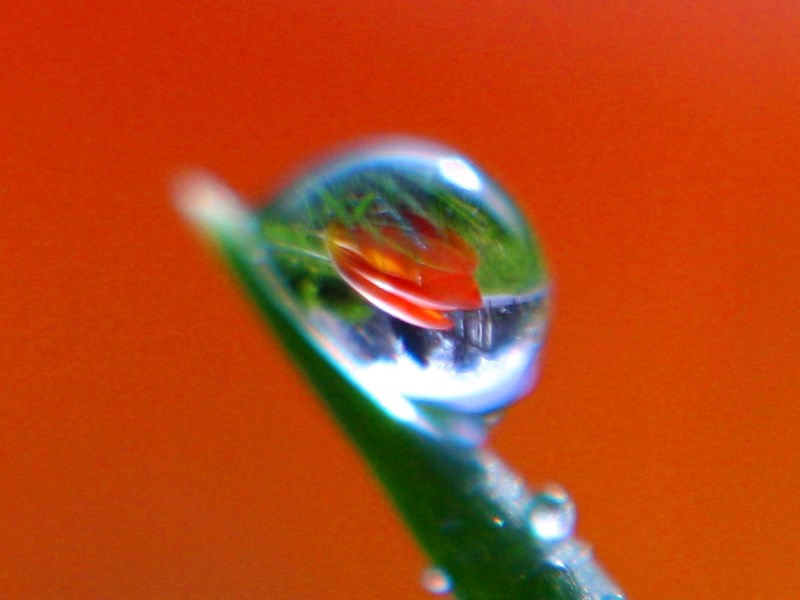In this captivating daytime close-up photo, a large, pristine water droplet delicately hangs from the tip of a slender, deep green blade of grass, suspended against a vibrant, cherry-red backdrop. Within this perfectly spherical droplet, an upside-down image of a fully bloomed red tulip with a green stem and leaves is crystal clear, magnifying and reflecting its stunning details. The red background, stretching diagonally from the bottom right to the upper left corner, suggests it's the petals of the tulip itself. The entire image, steeped in rich reds and greens, emphasizes the natural beauty and intricacy captured in this simple yet striking moment.